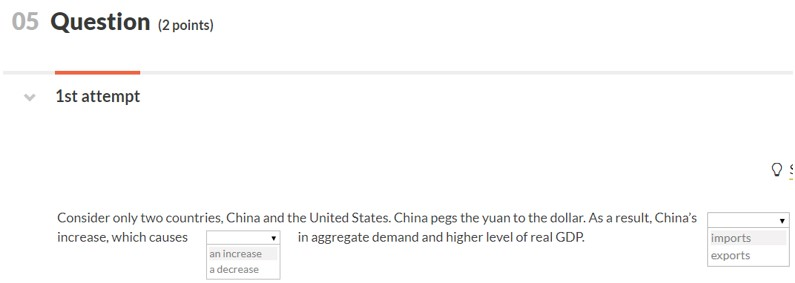The image is a screenshot from a website, featuring a white background. The specific website remains unidentified as there is no visible header or footer. The screenshot only captures a segment, focusing primarily on content from the left-hand side of the page.

At the top left, there is the number "05" in gray, followed by the word "Question" in bold. Beside this, in parentheses and regular font, it indicates "(2 points)." Beneath this is a gray line, with a portion of the line colored in red. Directly underneath the red segment, the text "First Attempt" is displayed in bold gray font. To the left of this, there is an inverted triangle suggesting the presence of a dropdown menu, likely for selecting an answer attempt option.

Slightly further down, the following instruction is given in gray text: "Consider only two countries, China and the United States. China pegs the yuan (Y-U-A-N) to the dollar. As a result, China's income, which causes," followed by a dropdown menu where the user can choose between "an increase" or "a decrease." The choice "increase" is currently selected. The sentence continues to say, "an aggregate demand and higher level of real GDP."

Additionally, it should be noted that earlier in the text, right after "As a result, China's," there is another dropdown menu, offering the choice between "imports" or "exports," which indicates another interactive selection area.

This screenshot appears to be from a page designed for an exam or exam practice, containing interactive question elements where users can select their answers from dropdown menus.